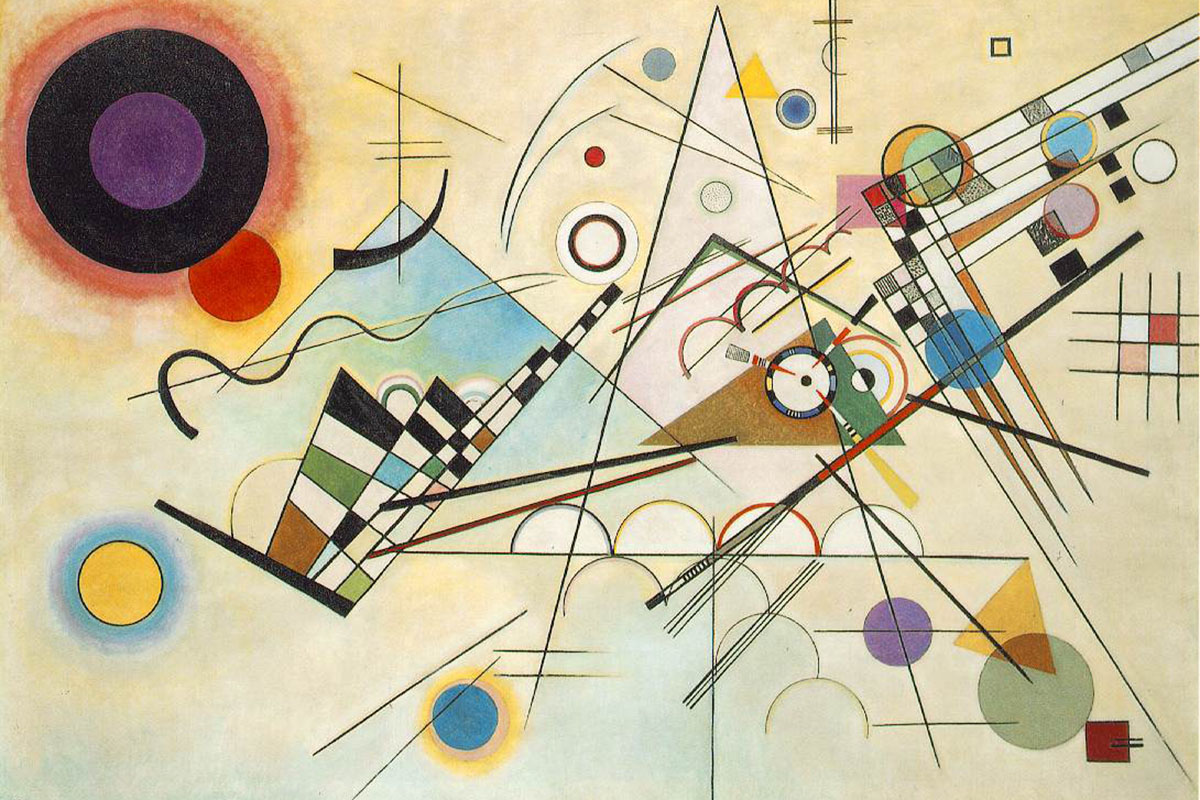"Composition 8 by Kandinsky is a colorful abstract modern art painting in landscape orientation. The image features a complex arrangement of geometrical shapes and intersecting lines. The background is a dirty cream color with a large, tall triangular shape outlined in black from top to bottom slightly off-center. 

In the top left corner, there is a black circle with a red halo and a purple circle inside it, accompanied by a smaller red circle on its bottom edge. Throughout the painting, there are numerous concentric circles in varying colors such as red, deeper red, yellow, blue, green, and white, along with black half-circles accented with blue, yellow, and red. 

The bottom left side has a yellow circle with a blue outline, and nearby, another yellow circle with a blue outline can be found towards the middle left. On the bottom right, various geometric shapes like a purple circle, a yellow triangle, a green circle, and a red square add to the composition. Scattered throughout are also blue, black, white, green, and brown boxes. 

In the center, a checked pattern resembles skyscrapers turned on their sides in layers of black, white, green, and brick color, with light blue triangular patterns behind them, adding to the dynamic feel with arcs, wisps, and squiggles in black creating movement. A gray, blue, and red object resembling a paintbrush and a multitude of thin lines, as well as lines with red, pink, and white boxes, intersect the composition, enhancing its modern, abstract essence."